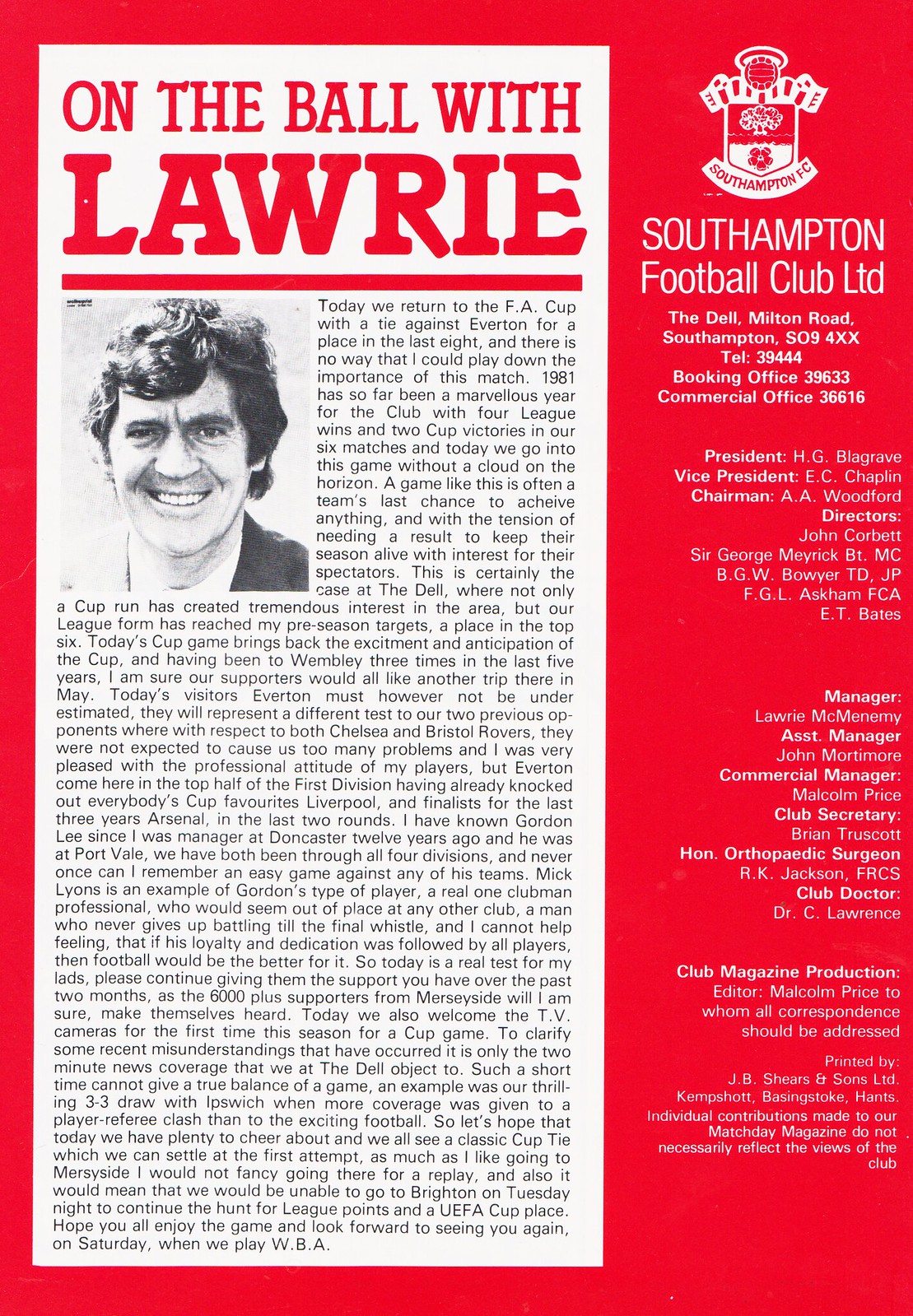The image is a newspaper or magazine clipping set against a bright red background, featuring an extensive article prominently titled "On the Ball with Lawrie." Positioned at the top of the left-hand side in red font, the title precedes an unbroken text block that delves into Lawrie's perspectives and experiences, including a significant mention of a match against Everton for a place in the last eight of the FA Cup and an account of Southampton Football Club's successful run in 1981 with four league wins and two cup victories. Accompanying the text is a black and white photograph of Lawrie, lending a personal touch to the article. The right-hand side of the clipping lists detailed information about Southampton Football Club Ltd, including their address at The Dell, Milton Road, Southampton, various office telephone numbers, and a complete enumeration of the club's officials, from the President, H.G. Blackgrave, to the Honorary Orthopedic Surgeon and the Club Magazine Production Editor.